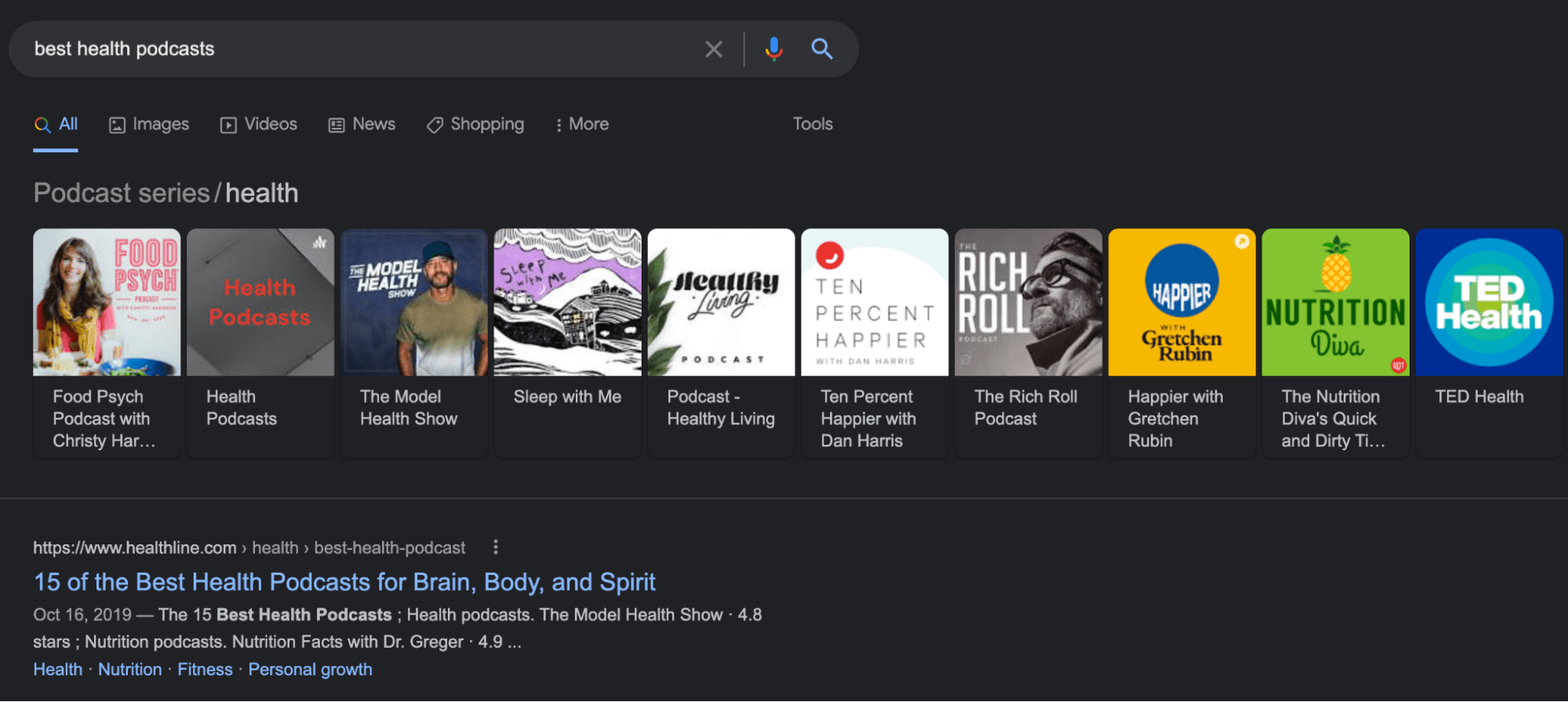The image showcases a Google search results page for "best health podcasts" with a distinctively styled search bar that includes a microphone and search icon. The query is highlighted and underlined in blue, emphasizing visibility. Below the search bar, Google’s navigation tabs—All, Images, Videos, News, Shopping, and More—along with Tools are prominently displayed.

The results feature a section titled "Podcast series," displaying several health-related podcasts. Notable mentions include:

- "Food Psych Podcast with Christy Harrison," 
- "Model Health," 
- "Sleep With Me," 
- "Healthy Living," 
- "10% Happier with Dan Harris," 
- "The Ritual Podcast," 
- "Happier with Gretchen Rubin," 
- "The Nutrition Diva's Quick and Dirty Tips," 
- "TED Health."

At the footer of the page, there's an article dated October 16, 2019, titled "15 of the Best Health Podcasts for Brain, Body, and Spirit," which lists top podcasts focusing on health, nutrition, fitness, and personal growth. The title and subject tags are highlighted in blue, making them stand out conspicuously against the background.